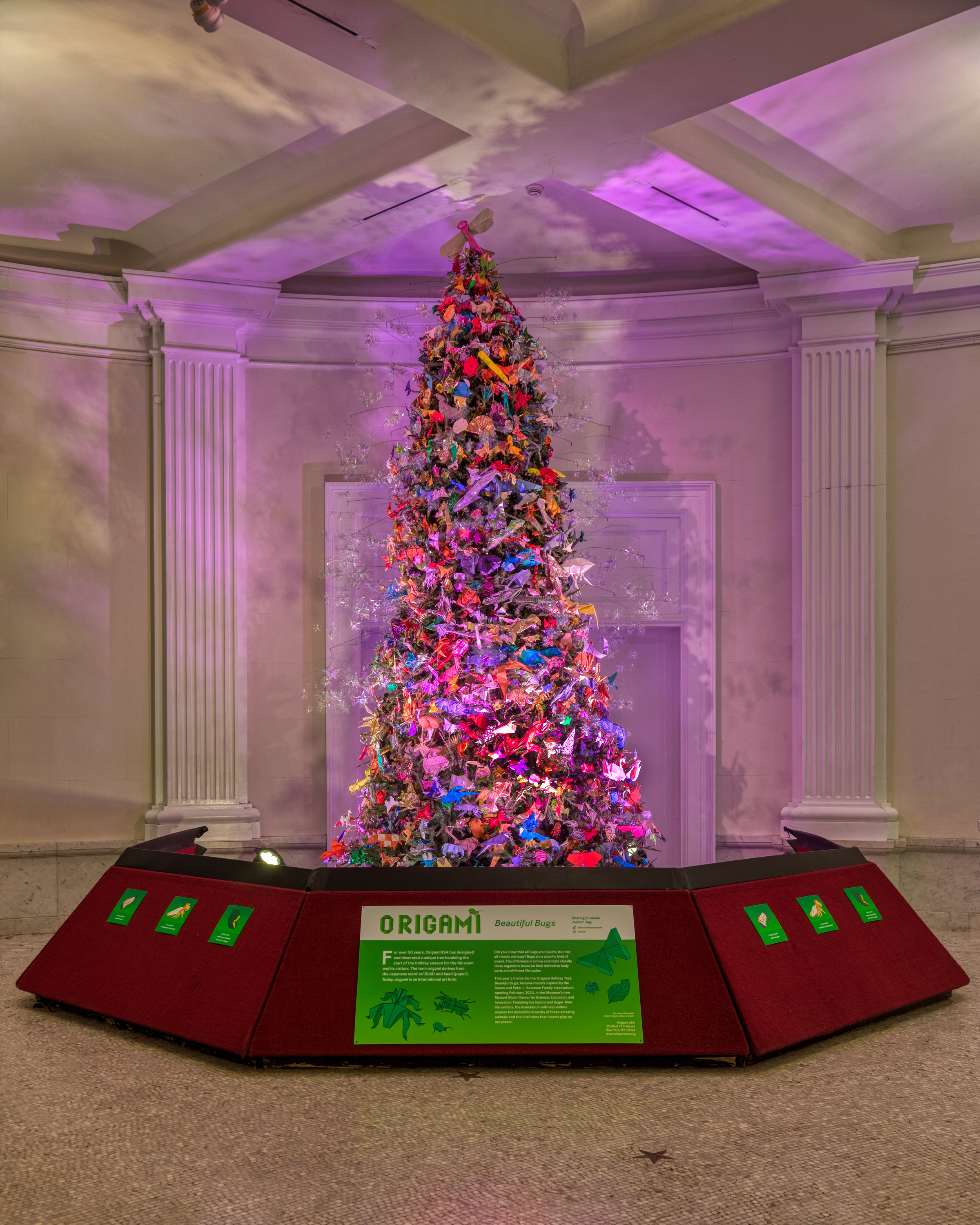This photograph captures a vibrant display of an indoor Christmas tree creatively adorned with numerous colorful origami figures in shades of orange, red, purple, and blue. The tree, standing out brightly in the center, is nearly completely covered by these intricate decorations, leaving hardly any green visible. It appears within a red angled partition, resembling an octagonal base with a gray tiled floor featuring a small brown five-pointed star inset. 

The partition, made of velvet-like red material, also showcases three green squares on each side, each adorned with unique emblems. Dominating the center is a large sign divided into two sections: a white top with green text reading "Origami Beautiful Bugs" and a green bottom featuring white text paragraphs with dark green origami figures arranged neatly around the text. The origami tree sits against a beige wall with two white striped columns extending upwards. A white squat doorway lies directly behind the tree, all framed under a ceiling with an X-shaped intersection of white beams, adding a structured aesthetic to the scene. This feast for the eyes is further enhanced by delicate thin branches with shiny translucent objects resembling snowflakes, adding a whimsical touch to this origami wonderland.